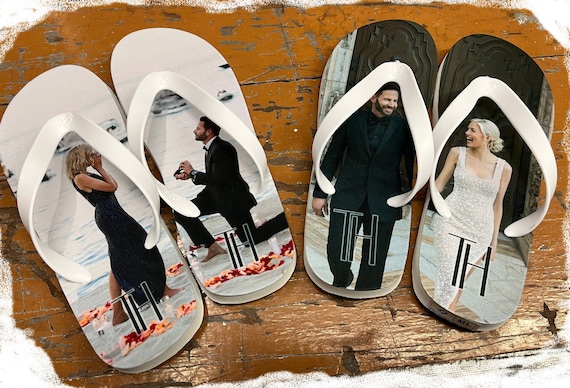The image depicts two custom-designed pairs of wedding-themed flip-flops. The first pair, predominantly white, showcases a romantic proposal scene. On the left flip-flop, a woman with blonde hair, dressed in black, stands with her hands to her face, reacting to a proposal. The right flip-flop features a barefoot man in a black suit, kneeling on a beach covered in rose petals, offering her a ring. The letters "TH" are visible near the heel area of these flip-flops. The second pair of flip-flops has a darker background but retains white straps, depicting the actual wedding day. The left flip-flop shows a man in a suit, while the right one illustrates a laughing woman in a sheer, white floral dress, gazing lovingly at him. Candles and rose petals accent the beach setting, adding to the romantic atmosphere.